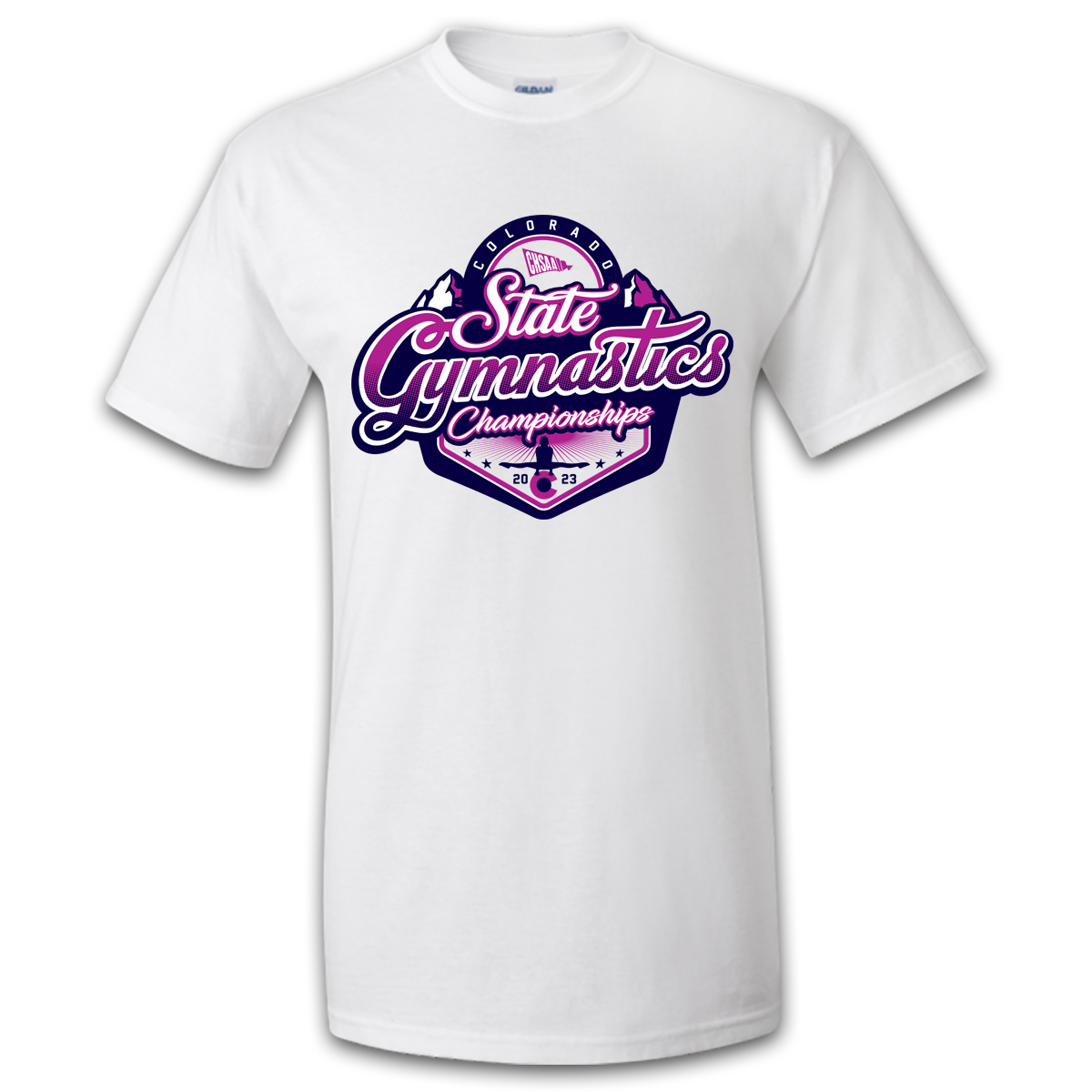In this detailed color photo of a white, crew-neck t-shirt against a white background with a subtle gray drop shadow, the design prominently features the Colorado State Gymnastics Championships for the year 2023. The text "Colorado" appears in white at the very top in a curved arch, while directly below, "State" is written in a cursive font with a white fill and a pink outline. The word "Gymnastics" is in the largest font size, showcasing an ombre color transition from pink to blue-purple. Beneath this, "Championships" is displayed in a smaller font. Complementing the text, there is a design element of a gymnast, rendered in black, performing splits across the letter 'C' in "Championships." Additionally, the layout includes some black stars, adding to the athletic theme. The overall composition looks like a mock image rather than an actual print on the t-shirt, emphasizing its conceptual design.